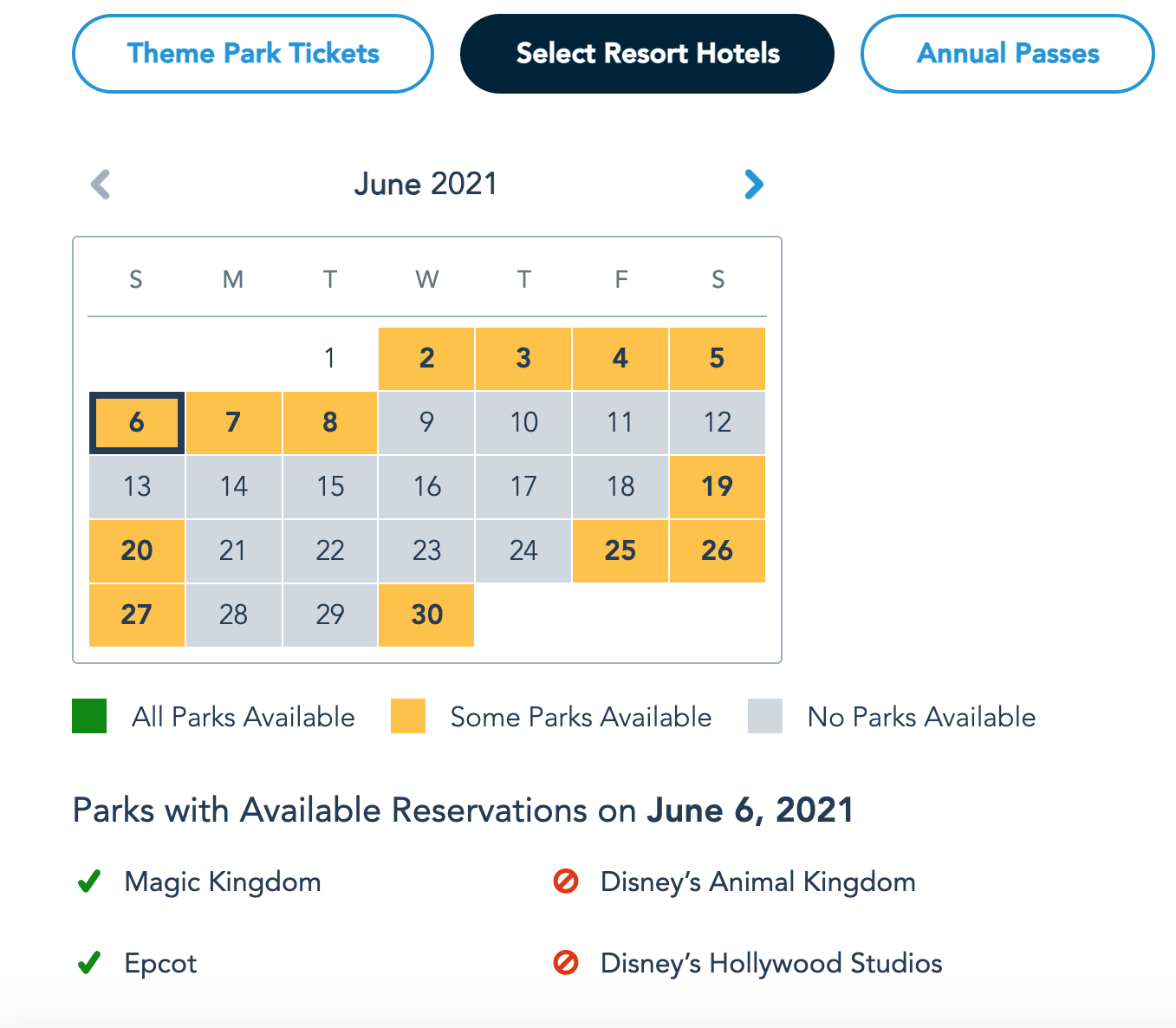The screenshot from the Disney World app or website features three selectable buttons at the top: "Theme Park Tickets," "Select Resort Hotels," and "Annual Passes." The "Select Resort Hotels" button is currently selected. Directly below these buttons is a calendar for June 2021. Navigation arrows are present, with the back arrow grayed out and the forward arrow highlighted in blue.

The calendar displays the month in a matrix from Sunday through Saturday. The availability for each day is color-coded: the 1st is in white, the 2nd through the 8th in yellow, the 9th through the 18th in gray, the 19th and 20th in yellow, the 21st through the 24th in gray, the 25th through the 27th in yellow, the 28th and 29th in gray, and the 30th in yellow.

Below the calendar, a legend explains the color codes: Green represents all parks being available, yellow indicates some parks are available, and gray signifies no parks are available. Further down, specific details for park availability on June 6th, 2021, are listed: Magic Kingdom and Epcot both show check marks, indicating availability, while Disney's Animal Kingdom and Disney's Hollywood Studios display stop signs, indicating no availability.